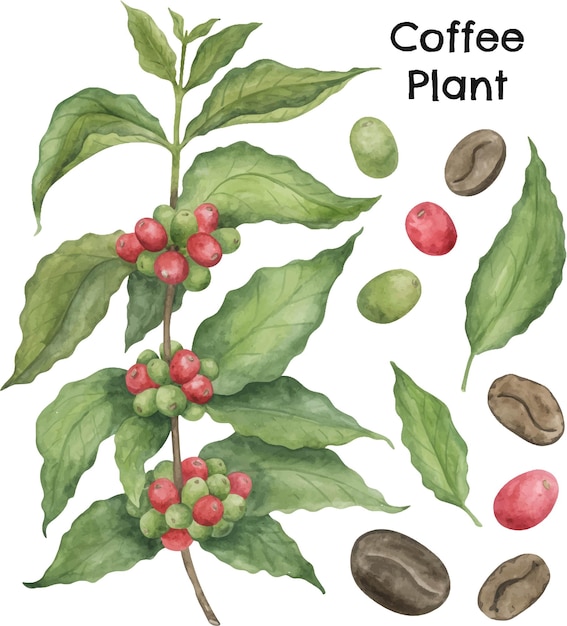This image is a hand-drawn and painted watercolor depiction of a coffee plant against a completely white background. On the left side, a long, central stem transitions from brown at the bottom to green at the top, with rows of vibrant green leaves extending from both sides. The plant showcases clusters of cylindrical berries or beans in varying stages of ripeness, with shades of green, faded red, and even brown. The red and green beans appear solid, while the brown ones exhibit a curvy line across the center. To the right of the main plant, there is a scattered collection of individual elements: more green and red beans, a couple of the vibrant green leaves, and a few brown coffee beans resembling the familiar roasted variety. At the top-right corner, the words "coffee plant" are inscribed in black lettering.